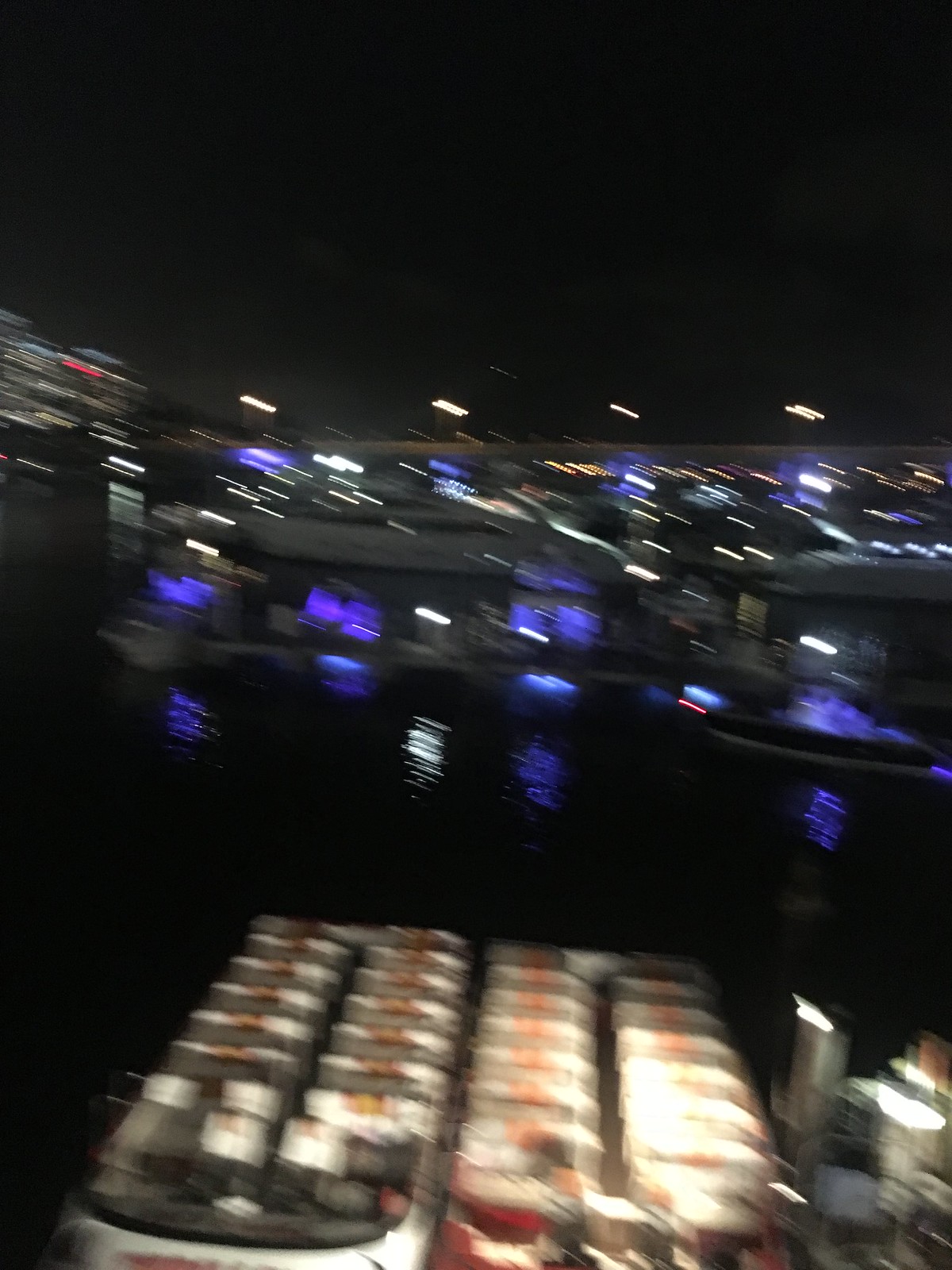A blurred, low-quality nighttime photograph captures an outdoor scene dominated by a dark sky with scattered distant lights. The image, taken from a waterfront perspective, shows reflections of white and blue lights on a body of water, suggesting ripples on the surface. At the bottom of the picture, two large boats with rows of white and red seats, possibly tour boats, are visible, casting illuminated reflections. The backdrop includes indistinct buildings, some featuring yellowish-white and blue lights, with one taller structure on the left adorned with red and white lights. The overall scene appears to be set in a marina or dock, accentuated by brown pillars and fleeting purple and gray blurs, which might be reflections or lighting artifacts.